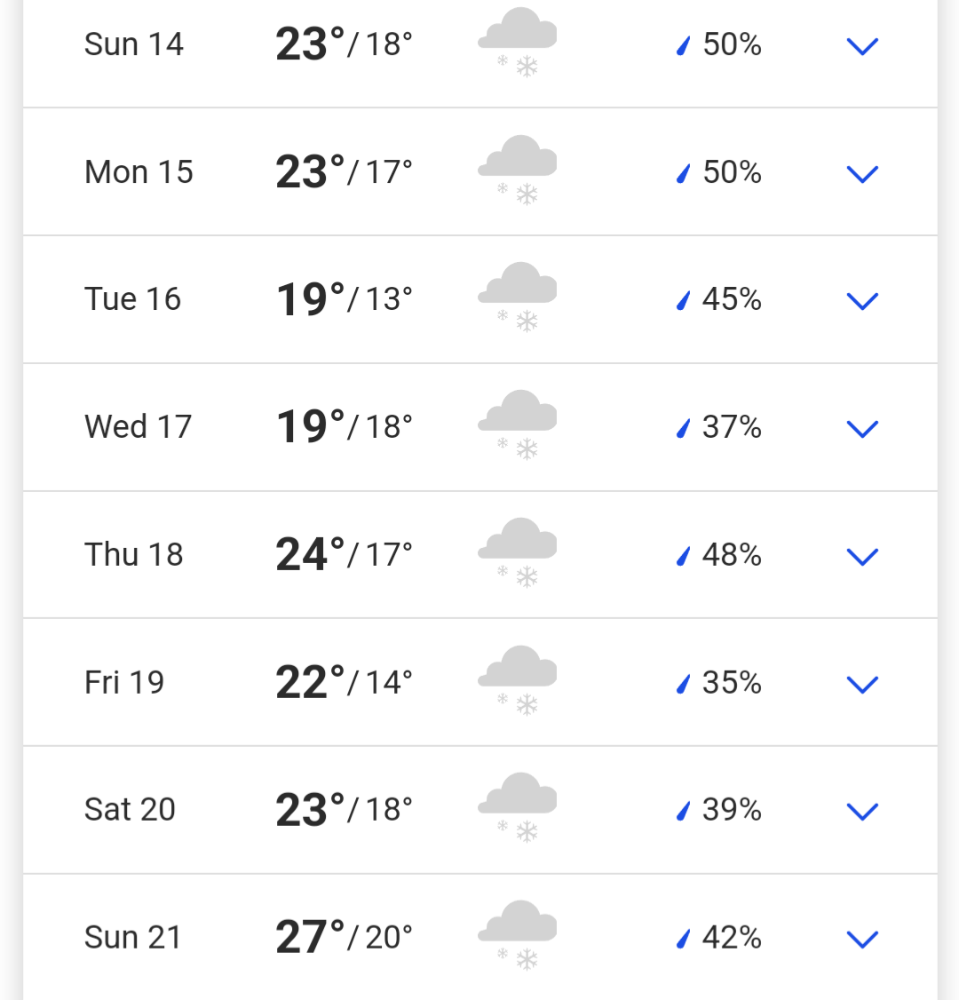This image showcases a weather forecast displayed on a smartphone screen. The forecast provides detailed weather information for a week, starting from Sunday and going through to the following Sunday.

- **Sunday, SUN 14**:
  - **Temperature**: 23°C / 18°C
  - **Symbols**: Cloud, Snowflake, Raindrop
  - **Probability of Precipitation**: 50%
  - **Additional Info**: Drop-down arrow for more details

- **Monday**:
  - **Temperature**: 23°C / 17°C
  - **Symbols**: Cloud, Snowflake, Raindrop
  - **Probability of Precipitation**: 50%
  - **Additional Info**: Drop-down arrow for more details

- **Tuesday, 16**:
  - **Temperature**: 19°C / 13°C
  - **Symbols**: Cloud, Snowflake, Raindrop
  - **Probability of Precipitation**: 45%
  - **Additional Info**: Drop-down arrow for more details

- **Wednesday, 17**:
  - **Temperature**: 19°C / 18°C
  - **Symbols**: Cloud, Snowflake, Raindrop
  - **Probability of Precipitation**: 37%
  - **Additional Info**: Drop-down arrow for more details

- **Thursday**:
  - **Temperature**: 24°C / 17°C
  - **Symbols**: Cloud, Snowflake, Raindrop
  - **Probability of Precipitation**: 48%
  - **Additional Info**: Drop-down arrow for more details

- **Friday, FRI 19**:
  - **Temperature**: 22°C / 14°C
  - **Symbols**: Cloud, Snowflake, Raindrop
  - **Probability of Precipitation**: 35%
  - **Additional Info**: Drop-down arrow for more details

- **Saturday, 20**:
  - **Temperature**: 23°C / 18°C
  - **Symbols**: Cloud, Snowflake, Raindrop
  - **Probability of Precipitation**: 39%
  - **Additional Info**: Drop-down arrow for more details

- **Sunday, SUN 21**:
  - **Temperature**: 27°C / 20°C
  - **Symbols**: Cloud, Snowflake, Raindrop
  - **Probability of Precipitation**: 42%
  - **Additional Info**: Drop-down arrow for more details

Each day on the forecast includes a combination of weather icons: a cloud, a snowflake, and a raindrop. Additionally, there's a percentage indicating the probability of precipitation and a drop-down arrow suggesting more detailed information is available.